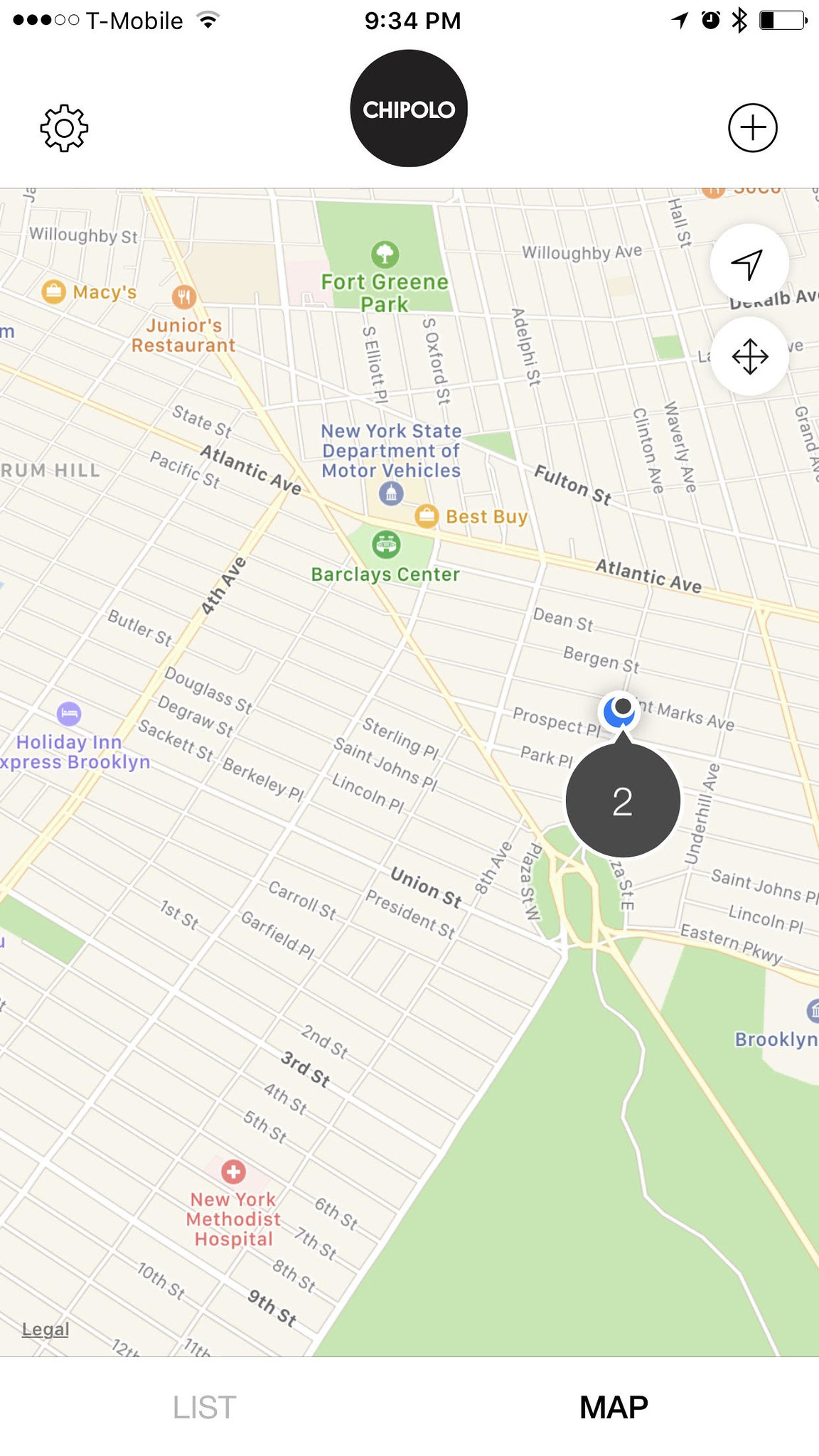This image is a detailed, interactive, digital map of a section of New York City, viewed on a computer. The map prominently features markers and symbols for various locations and landmarks, with controls that allow users to move and interact with it. Key locations highlighted on the map include New York Methodist Hospital, Macy's, Junior’s Restaurant, the Barclays Center, and the New York State Department of Motor Vehicles. There is also a green block indicating the location of Fort Greene Park. The streets visible on the map include 6th Street, 7th Street, Sterling Place, and Dean Street, suggesting that this is a densely developed urban neighborhood. Additionally, on the far right side of the map, Brooklyn is labeled. A notable marker, represented by a blue crescent symbol with the number "2" on it, is positioned around St. Marks Avenue and Prospect Place. The overall image captures a rich array of city infrastructure and amenities, offering insight into a vibrant and busy urban area.